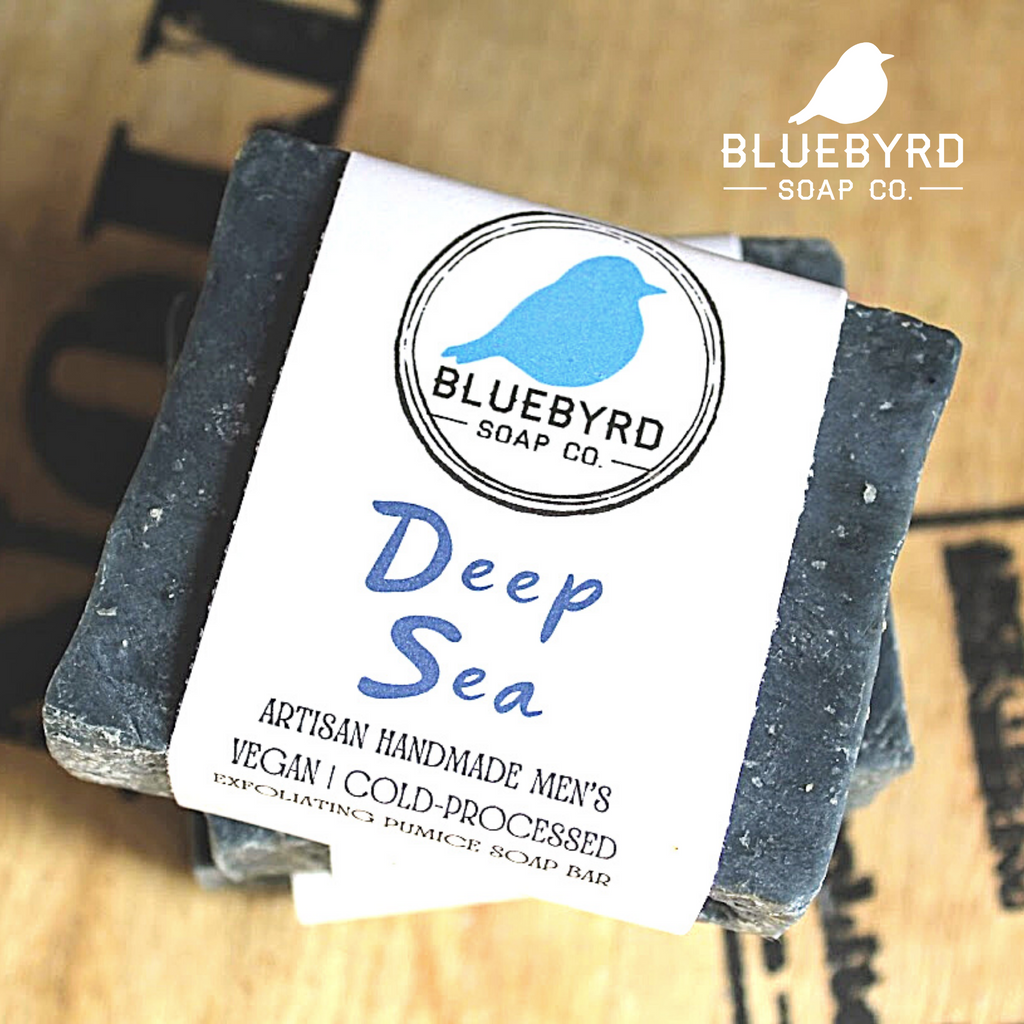The image is an advertisement for the Blue Byrd Soap Company, featuring a stack of three dark-colored, blackish soap bars with white specks, labeled as Deep Sea Artisan Handmade Men's Vegan Cold Processed Exfoliating Pumice Soap Bar. The soap bars are wrapped in a white paper with blue and black text. Prominently, "Deep Sea" is displayed in blue text at the center of the label. The top of the label features a logo with a blue bird, encircled by black rings, and the text "Blue Byrd Soap Company." Additionally, in the top right corner, there's a white version of the same blue bird logo with the same company branding. The entire display is set on a wooden surface, possibly atop a brown delivery box, against a background with some black text. The bird logo, reminiscent of an old Twitter bird, reinforces the branding throughout the advertisement.